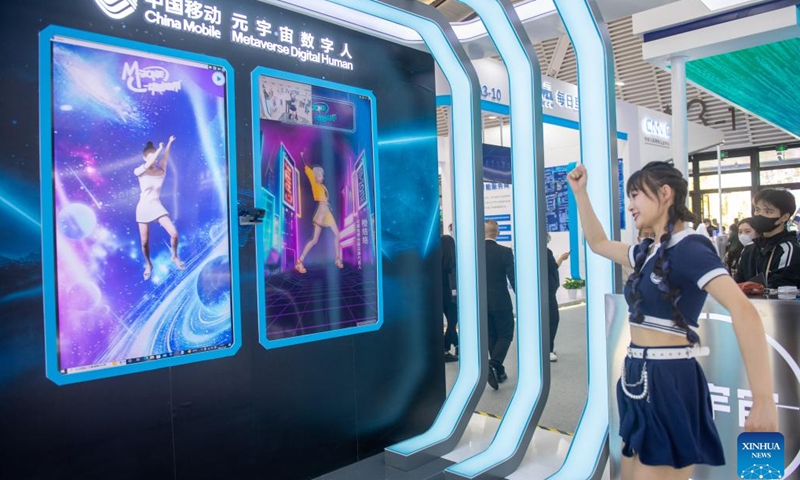The image is set in a public space, possibly an expo or convention in China, with a large screen labeled "China Mobile Metaverse Digital Human" in the top left corner. The photo, credited to ZUNANEWS (Xinhua), depicts a young woman with braided hair wearing a navy blue and white sailor-style schoolgirl uniform - a crop top with white edges and a blue skirt with a white belt. She is standing in front of a futuristic kiosk, with neon whitish-blue lights and a pad on the floor, appearing to play a virtual reality dance game. The screen shows two digital avatars dancing: one on the left amid blue and pink spacey visuals and another on the right in a neon pink and blue cityscape setting. The woman mimics the dance movements of the avatars, her focus intent on the screen. Behind her, a few masked onlookers watch, and there are several white booths visible in the background, indicating a busy, public location filled with people.